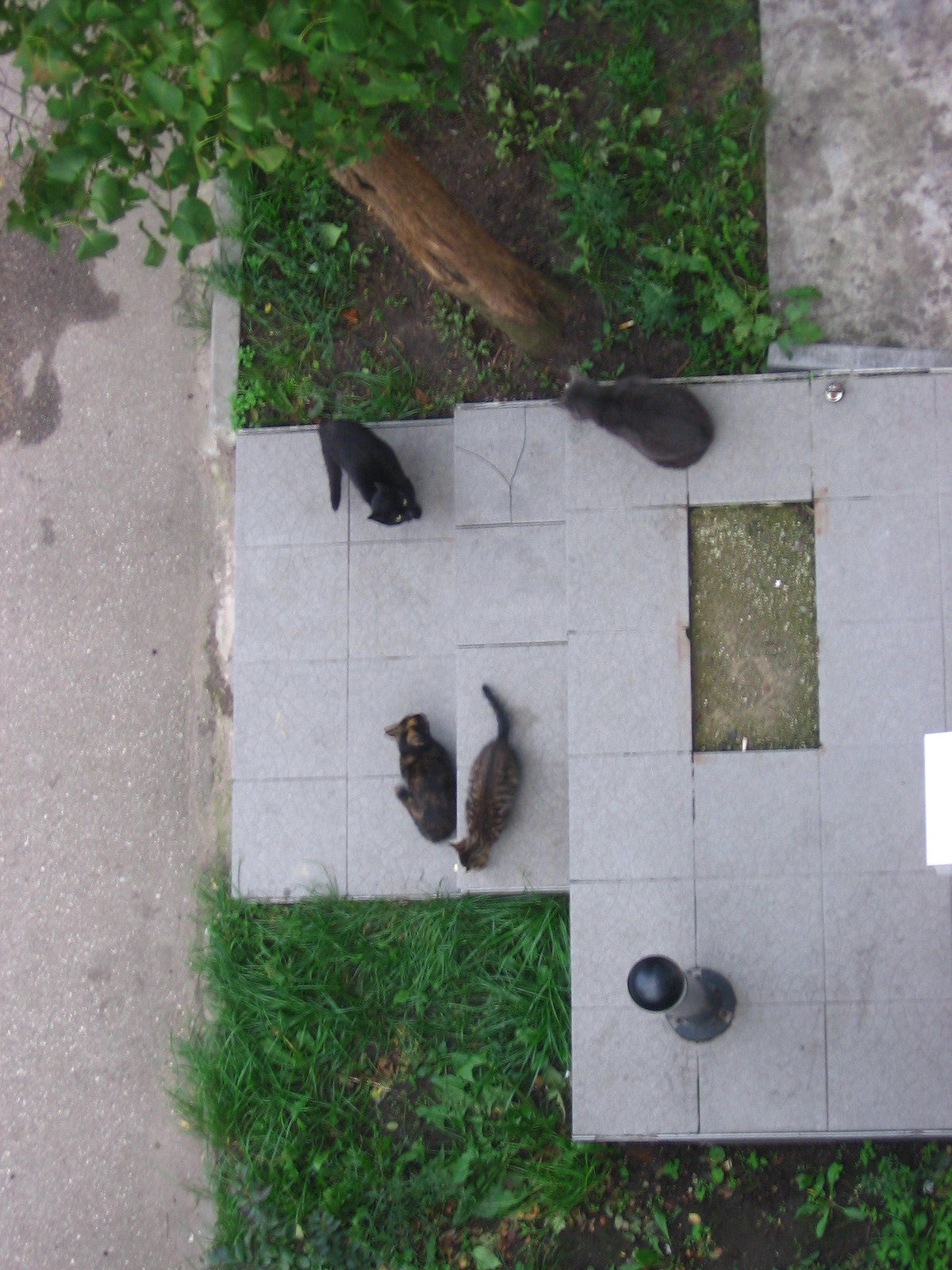This overhead view captures a scene of four cats lounging on concrete steps surrounded by patches of overgrown grass and a small tree. The steps ascend to a rectangular landing with bare, dirt-filled space amid a concrete boundary. On the left side of the image, part of a gray asphalt road is visible. The feline arrangement on the steps is notable: on the lower steps, a gray cat lies on its back with paws up, next to it is a dark gray cat gazing upward as if planning its next leap. Above them, another brown-gray cat stretches out with its tail extended, seemingly fixated on something below. Topping the steps, a black cat stares intently at the person taking the photograph. The left and right edges of the steps are framed by encroaching grass, with a small tree nestled in the greenery to the right of the steps.